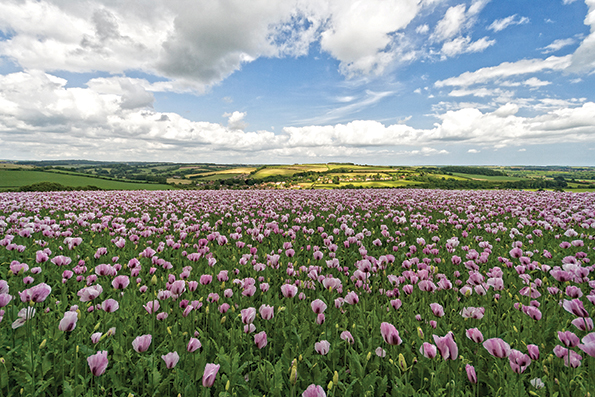This photorealistic outdoor image captures an expansive field filled with countless vibrant flowers, primarily purple tulips that extend as far as the eye can see. The scene is dominated by the lush greenery of the tulip leaves and stems, interspersed with patches that reveal the rich, tan dirt beneath. In the far background, a picturesque valley unfolds, featuring rolling green hills and farmland, with the occasional house dotting the landscape. Above, the sky is a bright and clear blue, adorned by clusters of white, puffy cumulonimbus clouds. The sunlight gently beams down, illuminating the scene with a soft glow, enhancing the stunning contrast between the colorful flowers below and the serene sky above.